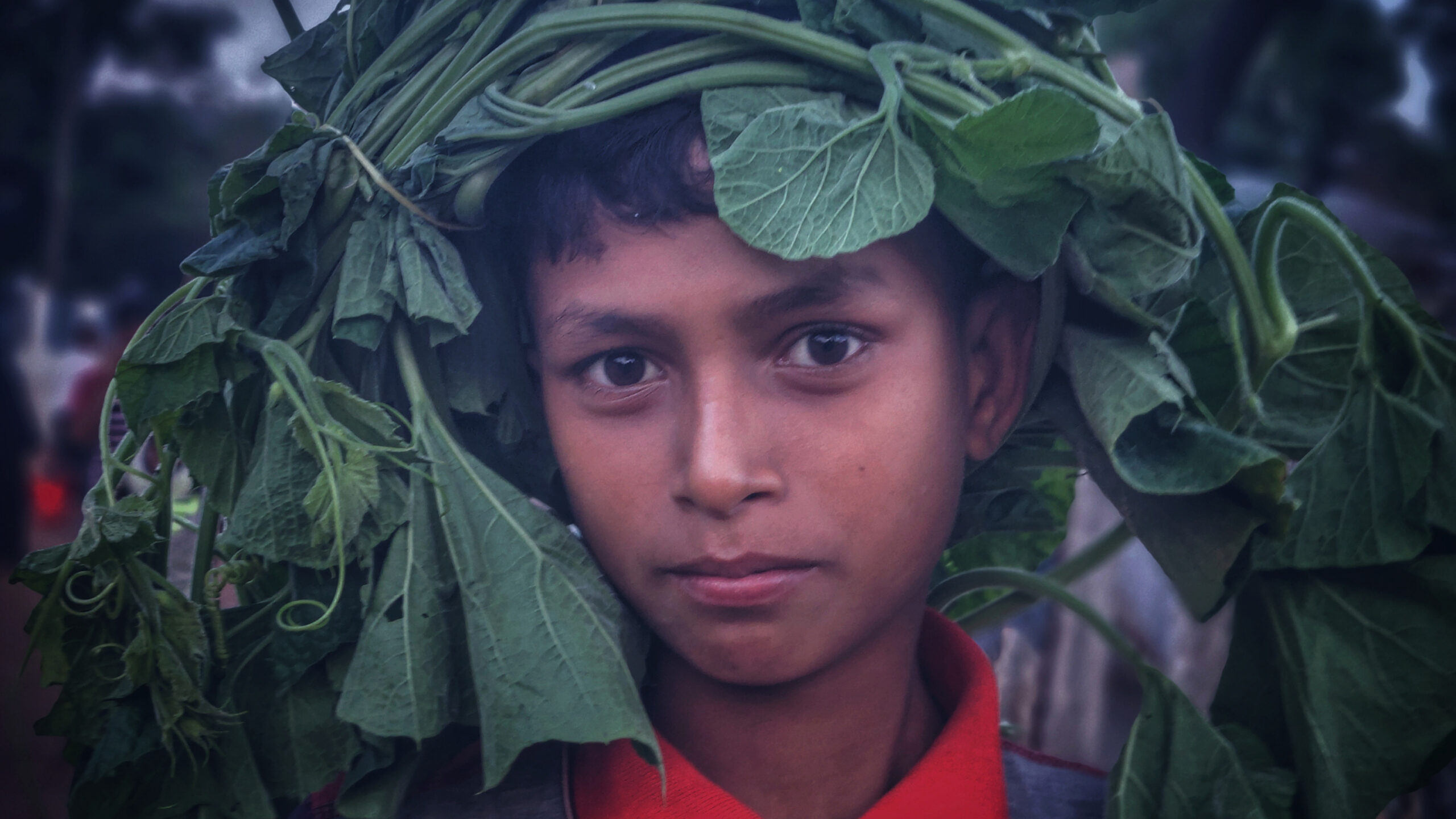This real-life photograph captures a young boy, estimated to be around 8 to 11 years old, with dark skin, possibly of Hispanic, Indian, or Southeast Asian descent. The image is an up-close shot focusing on his face and neck, giving prominence to his large, dark brown eyes and black hair. He wears a red collared shirt with hints of blue and dark red from another garment over it. Notably, his head is adorned with a unique headdress made of plant vines, likely from a squash or similar vegetable plant, featuring large green leaves and curly tendrils. The vines cascade from one shoulder to the other, enveloping the space around his head. The background is blurred and dark, possibly hinting at trees and a shadowy figure, but remains indistinct. The boy gazes directly into the camera, his expression composed and his mouth closed, adding a captivating and intriguing element to the portrait.